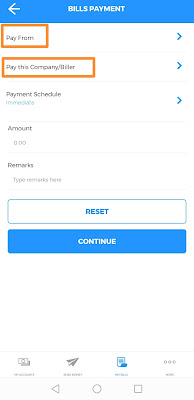This image appears to be a screenshot from a website dedicated to bill payment. The top portion, around an inch in height, features a light blue background. To the left side of this area is a large white arrow pointing to the left. Centrally located and displayed in bold, capitalized white letters are the words "BILLS PAYMENT." 

Below this, down to about an inch from the bottom, the background turns white. On the left side, near the top, there is an orange square with black lettering that reads "PAY FROM." To the right, there is a blue greater-than sign (>) pointing rightward. Below this, more text appears, reading "Pay this company / [blurry text, appears to be five letters]," enclosed in a thick orange border.

On the right side of the section, there is another blue greater-than sign pointing to the right. Underneath, the text "PAYMENT SCHEDULE" is in black, followed by "IMMEDIATELY" in blue, flanked by another greater-than sign.

Further down, the text "AMOUNT," followed by another segment labeled "REMARKS" with the prompt "Type remarks here" is visible. Beneath this is a white tab with a blue border, displaying the word "RESET" in bold, capitalized blue letters. Below this is another tab that reads "CONTINUE" in bold, white letters.

At the very bottom of the image, there appear to be several icons: a camera icon, a search icon, and a somewhat unclear label for each, ending with a blue square and three ellipses. Lastly, at the very bottom, left side, there is a set of symbols typical of a phone interface: a left-pointing triangle, a circle in the center, and a square on the far right.